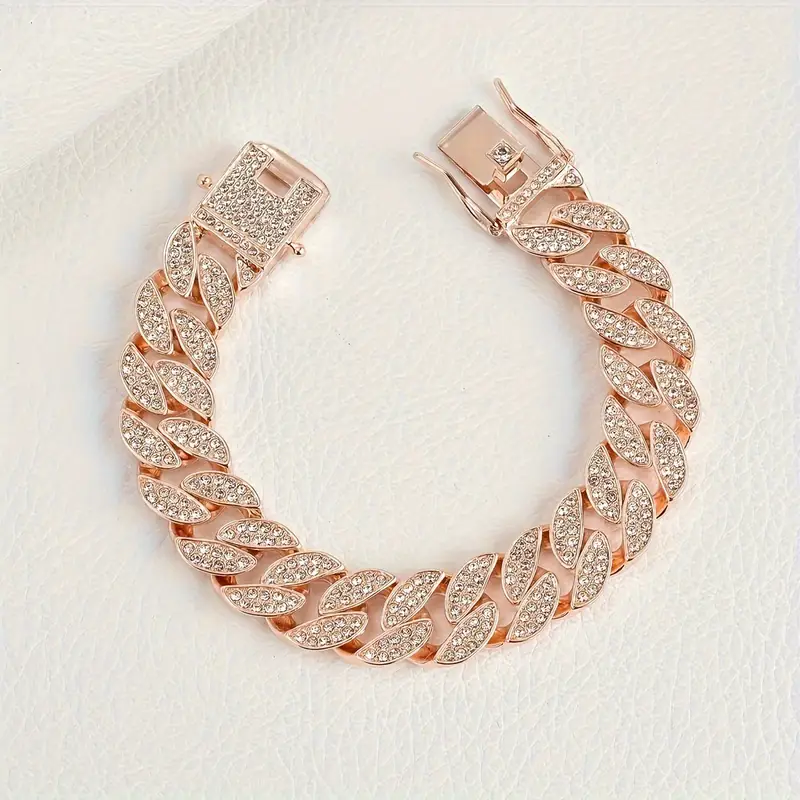An up-close image reveals a rose gold bracelet placed against a white, textured, leather-like background. The bracelet, curved in a circle with its clasps unclasped at the top, showcases an intricate design featuring pairs of leaf-like shapes that run along its entire length. Each leaf shape, slightly slanted and filled with approximately eight clear, sparkly stones—likely diamonds or possibly high-quality imitation gems—adds a luxurious touch. The detail and craftsmanship are highlighted by the diamond-encrusted clasp on the left, which appears designed to secure the other end with a pointy latch mechanism, ensuring a firm closure. The elegant pattern of elevated sections holding these sparkling stones continues uniformly around the bracelet, emphasizing the exquisite combination of rose gold and diamond-like brilliance.